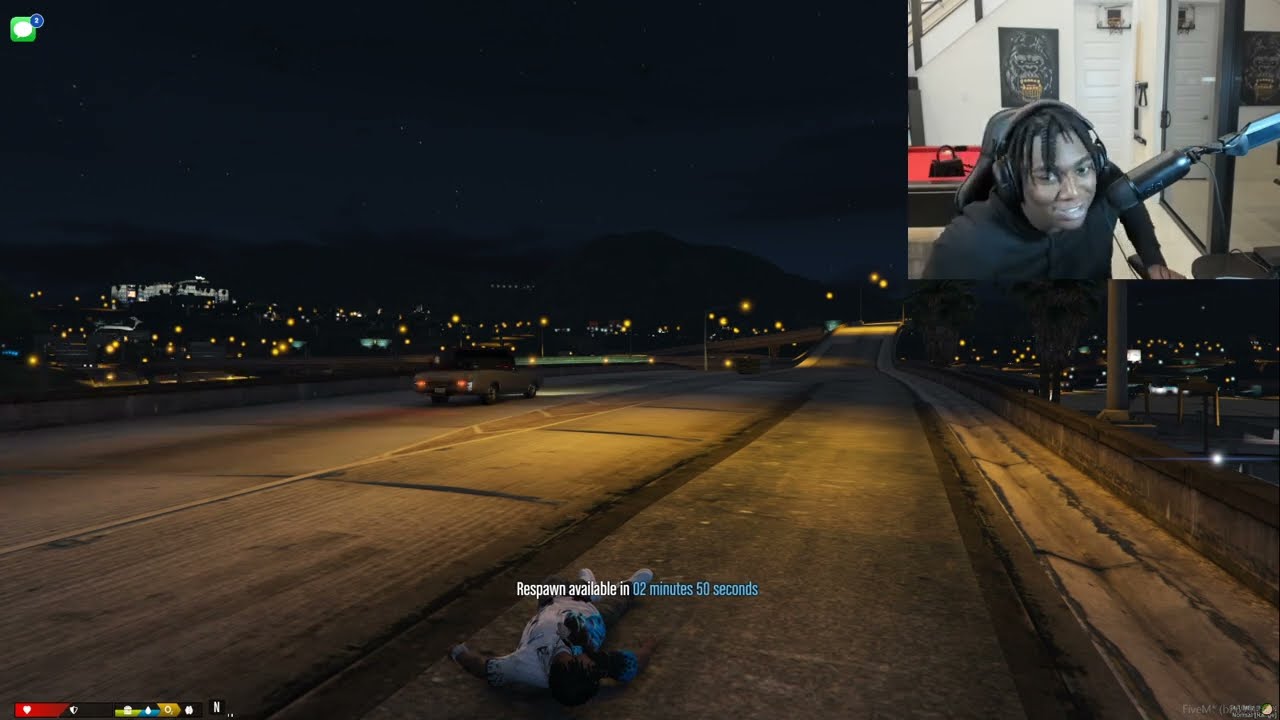The image is a frame from a live stream or YouTube video of someone playing a video game. In the top right corner, there is a small box showing a young man sitting in a leather chair with a headset on, talking through a microphone attached to a mic arm. Behind him, there's a poster of King Kong and a red pool table, giving the impression he's in a basement. The game scene takes place on a wide highway at night, with city lights and shadowy mountains visible in the distance. A single car drives on the left side of the road. Lying in the middle of the highway is a human figure, seemingly dead, wearing a bloodstained white shirt. Text on the screen reads, "Respawn available in two minutes 50 seconds," suggesting the character will return to the game shortly.